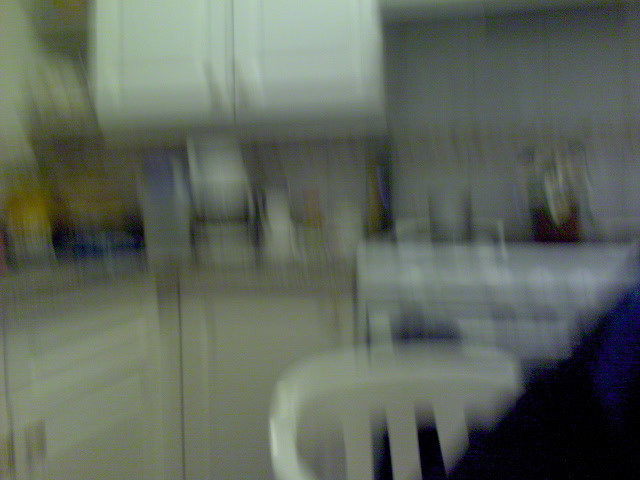This photograph, taken in a hurried or unsteady moment, offers a blurry glimpse into a cozy kitchen corner. The focus is on the intersection of counters and cabinets, where white cabinetry adorns both the upper and lower sections. The countertop, with its brown or tan marbled finish, is dotted with various containers, hinting at daily kitchen activities. To the right, a white stove with matching knobs subtly stands out. In the foreground, partially obscuring the stove, is a white chair. Though a person appears to be seated in the chair, only a dark, indistinct shape, presumably their back or torso, is visible, adding a sense of mystery to the scene.